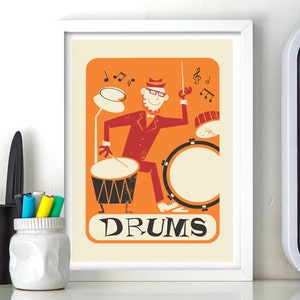The image features a cartoonish caricature of a bearded man playing the drums, prominently displayed in the center within a white wooden frame, which is bordered by a cream inner edge. The background of the drawing is bright orange. The cartoon character, dressed in a red suit and glasses, is depicted with a white face and a beatnik-like appearance from the 1950s. He is playing a black drum with his right hand and raising another drumstick with his left hand. Additional drums, including a black-edged circular one, and music notes are present around him. Beneath the illustration is a rounded rectangular white text box with the word "drums" written in large black letters.

The framed artwork leans against a wall, positioned either on a white tabletop or a shelf. To the left of the frame, there is a white jar holding three highlighters in green, yellow, and blue. Next to the jar, a black cylindrical object, possibly a stapler, leans against the wall. The image captures a mix of vibrant colors with a dominantly orange, red, and black color scheme, accented by the clean white frames and tabletop to create a vivid display.